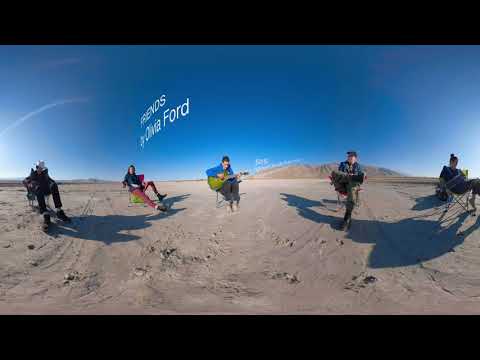This is a detailed panoramic photo capturing a band of five friends seated in lawn chairs in a sandy desert landscape. In the clear, bright blue sky above, white text floats, reading "FRIENDS" in all caps with "by Olivia Ford" in smaller, capitalized initial letters. The band members, positioned from left to right, are somewhat distant, making it difficult to identify all the instruments they are playing. Notably, one member in the center is wearing a blue hat and playing a green guitar, while another appears to be holding an accordion. The ensemble includes at least one female member on the far right side, with the rest likely being males. The desert setting features a rocky outcropping or a mountain in the background, and the foreground shows some prints or markings in the sand. The photo has slight distortions, giving a sense of an expansive, open space under a clear sky, with just a hint of a vapor trail from a plane.